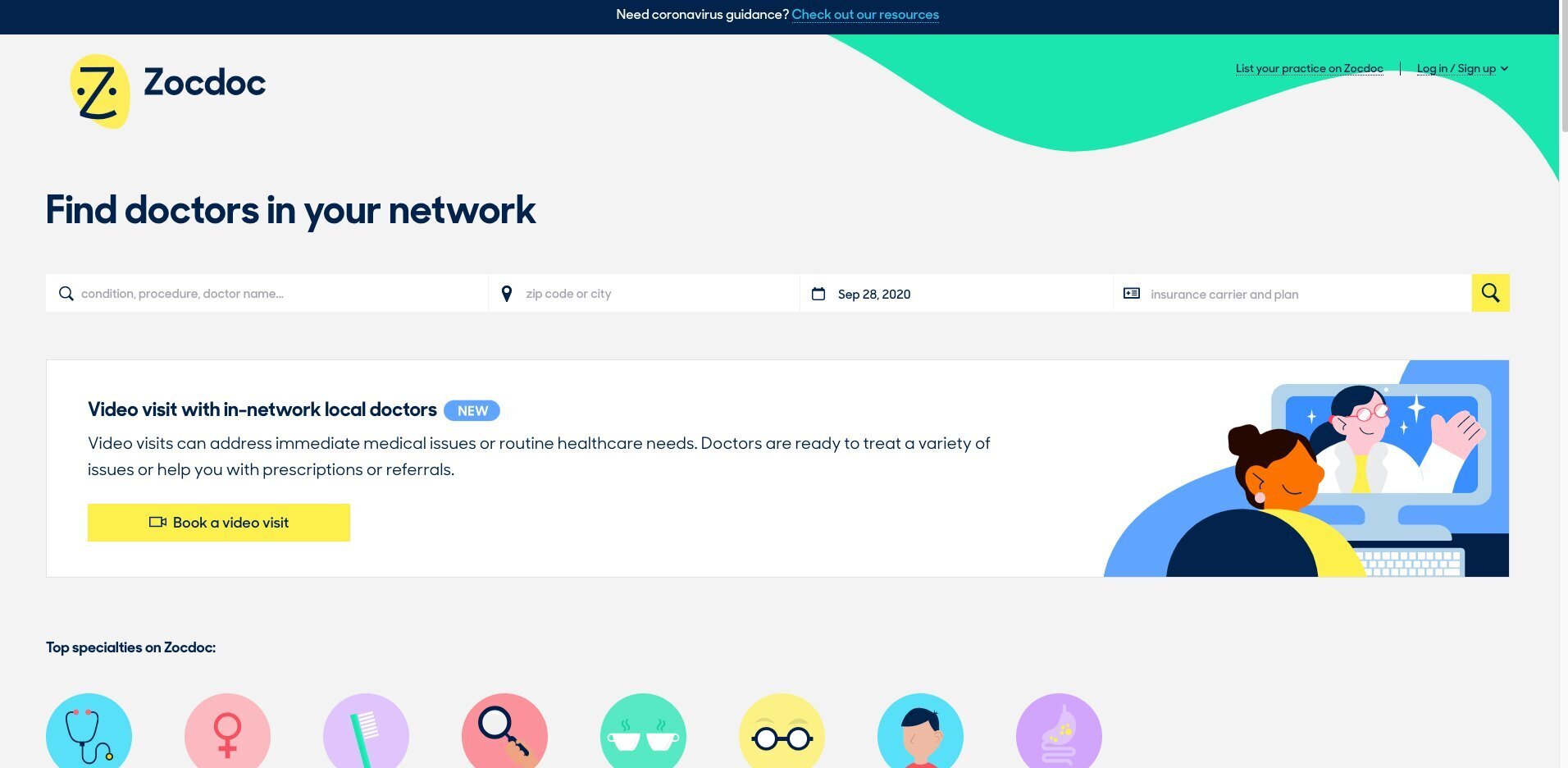This detailed description is of an illustration for Zodok. The primary feature is a yellow oval resembling a face with two eyes and a prominent 'Z' in the center, representing the Zodok brand. The backdrop is predominantly white unless specified otherwise.

Prominently, the phrase "Find doctors in your network" is displayed in bold navy blue text. Below this, information categories such as "Condition prognosis," "Doctor notes," and search fields for "zip code or city" are included. It also shows the date, "September 2020", along with fields for insurance carrier and plan, adorned with a small emblem. This entire section is encased in a white box.

Specifically, the phrase “video visit within network local doctors new” stands out in bold navy blue font, indicating the availability of video consultations. The accompanying text explains that "Video visits can address immediate medical issues or routine healthcare needs. Doctors are ready to treat a variety of issues or help you with prescriptions or referrals,” emphasizing the service's utility.

Towards the bottom, a bright yellow box invites users with a call-to-action: "Book a video visit."

On the right side of the illustration, a hand-drawn scene depicts a female doctor with a stethoscope, waving to a woman seated in front of her computer screen, signifying a virtual consultation setup.

At the bottom, a section titled "Top Specialties" features icons including a stethoscope (likely indicating general health or pregnancy), a toothbrush (suggesting dental care), a magnifying glass, two steaming coffee cups, eyeglasses, a child, and an illustration of the stomach and intestines, hinting at various medical specialties and services provided.